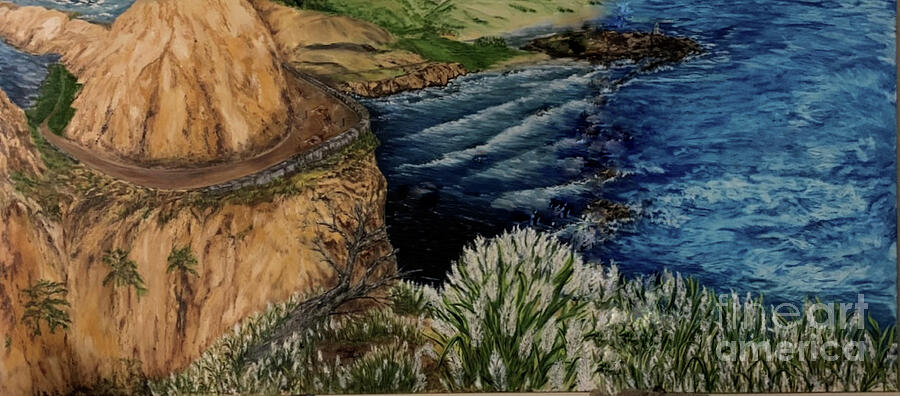The detailed etching captures a scenic shoreline dominated by tall, steep cliffs of a light brown hue, leading down to a deep blue, wave-filled ocean. At the base of the cliffs, a serene cove with dark brown rock lines cradles the water, where waves crash against the shore. Atop the cliffs, a dirt road winds around a domed rock formation, bordered by a stone wall that overlooks the ocean. The greenery spread across the scene includes tall green plants with fuzzy white flowers on the right side, suggesting a natural, untamed beauty. The artwork is delicately signed "Fine Art America" in white writing in the lower right corner, subtly acknowledging the creator.